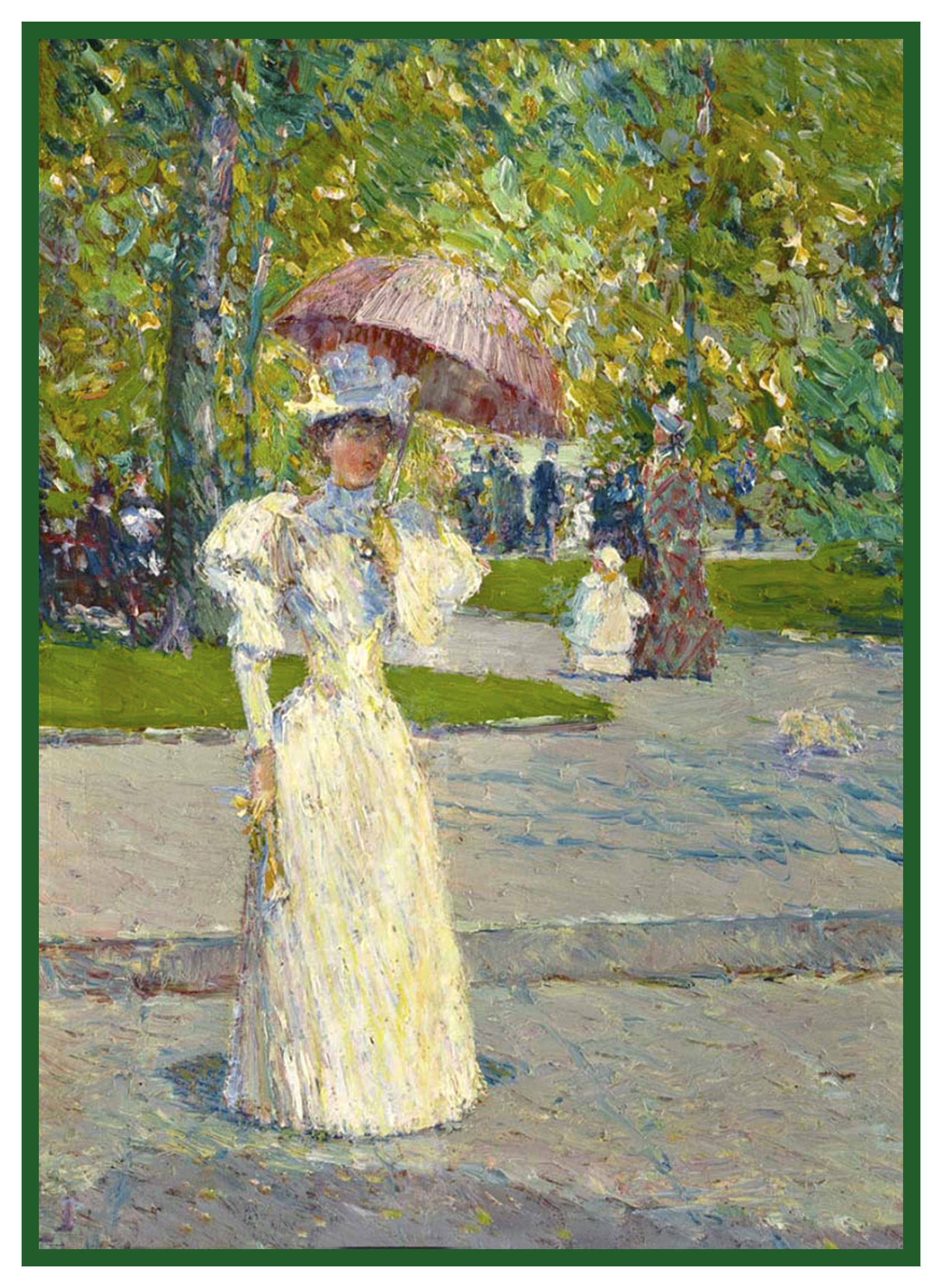The image captures an exquisite outdoor scene from the 1800s, painted with either oil or pastel on canvas. With natural daylight illuminating the scene, the vertical rectangular painting is encased in a thin green border that enhances its vibrancy. The setting is a public park teeming with lush greenery, where numerous trees tower in the background. The park's expansive green lawns and winding walkways are peopled with men, women, and children clad in period attire, creating a lively, communal atmosphere. 

Central to the composition is a woman in an opulent, floor-length white gown adorned with poofy shoulders and upper sleeves, exuding an air of formality. She wears an ornate white hat and carries a reddish umbrella to shield herself from the sun, adding a splash of color to her elegant ensemble. To her right, a mother and child, the latter dressed entirely in white, complement the scene. Nearby, another figure in a stunning yellow gown—highlighted by a floral bracelet and a bonnet—strolls gracefully, holding a pinkish umbrella. This intricate, genteel tableau is brilliantly captured, making the painting a beautiful homage to its time and setting.